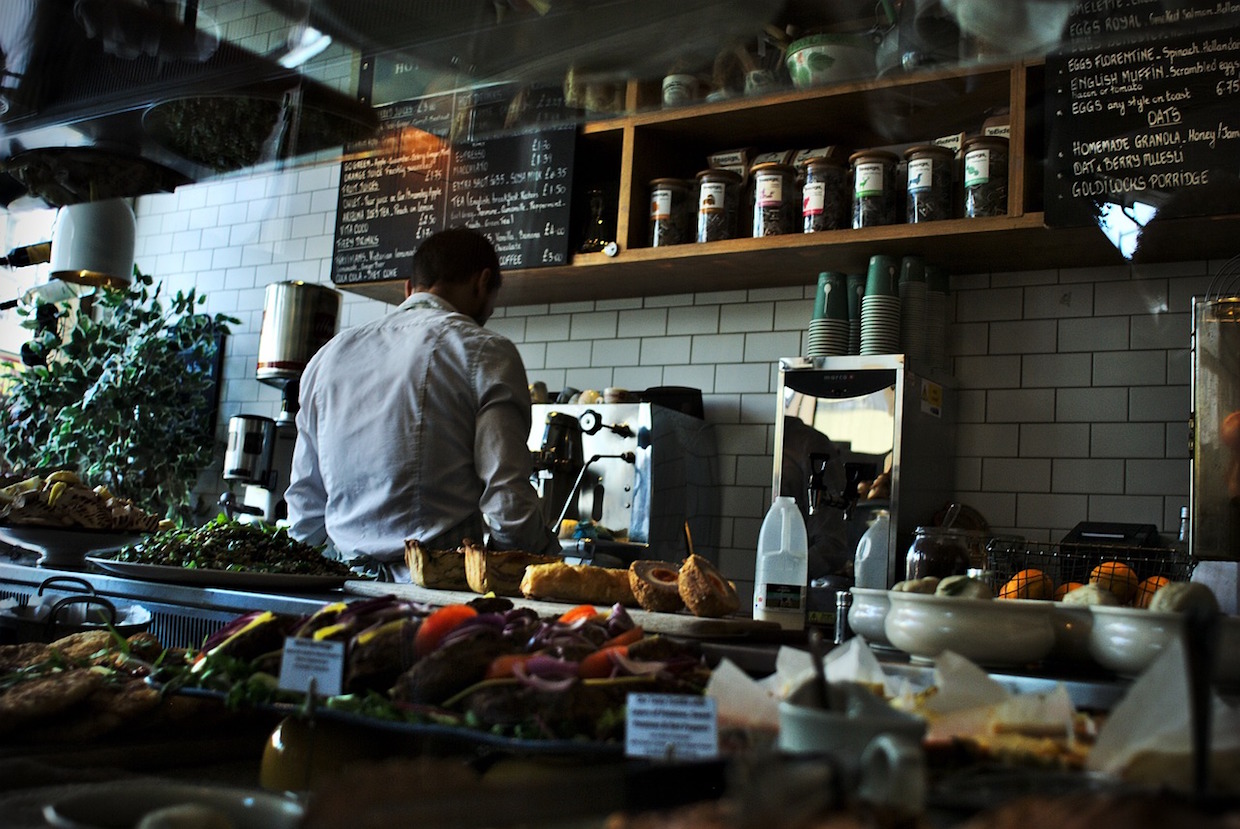This image captures the bustling scene of a coffee shop or cafe, filled with a vibrant array of food and drink preparations. The focal point is a man, seen from behind, standing at the counter working with several stainless-steel machines, including a coffee machine prominently in use. Cups are neatly stacked on an adjacent machine, possibly an espresso machine or a coffee bean grinder. To his left, a half-gallon plastic container of milk is visible amidst a plethora of jars and containers that hint at various condiments and syrups, though their exact contents are indistinguishable due to the image's dim lighting.

The counter itself stretches from left to right, laden with diverse food items. Among them are a variety of baked goods, including bagels, and an assortment of toppings like olives, onions, and possibly some cream cheese and lox. Though the labels on these items are hard to discern, they contribute to the rich detail of the scene. Above the counter, the background is decorated with white subway tiles and two blackboards, both with handwritten menus, sandwiching a wooden shelf. The shelf displays seven canisters of coffee or tea, each adorned with colorful labels.

Further adding to the cafe's charm, the blackboard to the right lists specific offerings such as oats, homemade granola, berry muesli, and a uniquely named Goldilocks porridge. Below a secondary shelf, there are fresh salad greens, bread, and various fruits arranged with care. Despite the overall dark tone of the photograph, the image vividly conveys a cozy, rustic atmosphere bustling with the preparations of delectable treats and beverages.